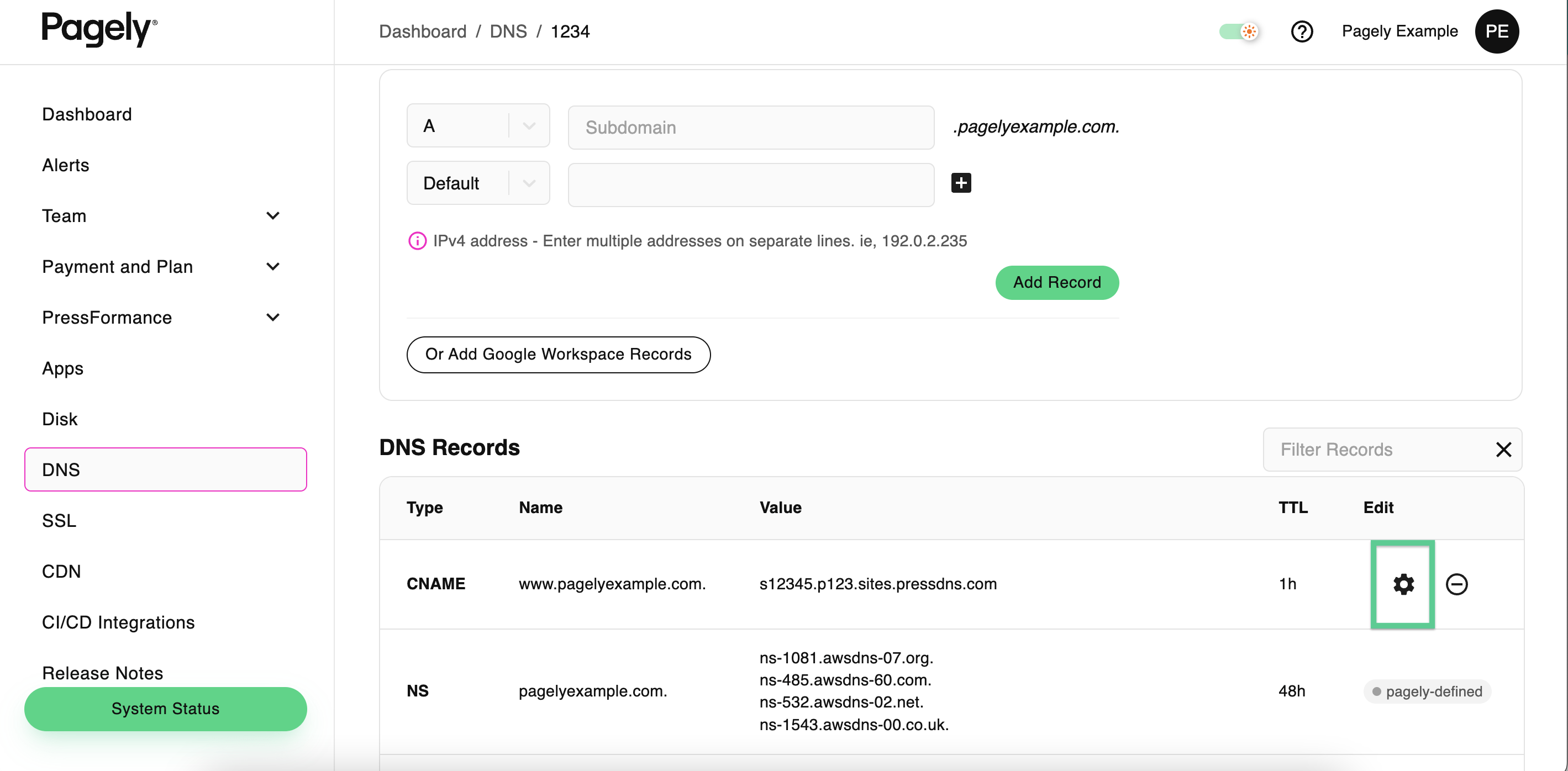The image is a detailed screenshot of a web page dashboard for Pagely, characterized by a clean white background. In the upper-left corner, the company name "Pagely" is displayed prominently in a black, sans-serif font, paired with a likely registered trademark symbol next to the 'Y'. This text occupies the header section of the page. 

To the right of the header, a breadcrumb navigation trail reads "Dashboard / DNS / 1234", guiding the user through their current location within the dashboard. The upper-right corner contains the text "Pagely example" beside a black circle featuring the white initials "P-E".

On the left side, a vertical sidebar menu is presented in black font, comprising the following options: "Dashboard," "Alerts," "Team," "Payment and Plan," "Press Formats" (listed as one word), "Apps," "Disk," "DNS," with "DNS" being highlighted with a pink rectangle, and further down, "SSL," "CDN," "CI/CD Integrations," and "Release Notes." Notably, at the bottom of the sidebar, a green rectangular button with rounded corners and black text reads "System Status".

Occupying the main section of the page is a configuration area for website settings. At the top of this section is a large letter "A," suggesting a subsection for subdomain configuration due to the accompanying label "Subdomain." Below, a prominent headline states "DNS Records and Type," listing different record types like "CNAME" and "NS" (Name Servers). In the top-right, a small circle with notches hints at additional settings or a refresh button, encircled by a green rectangle.